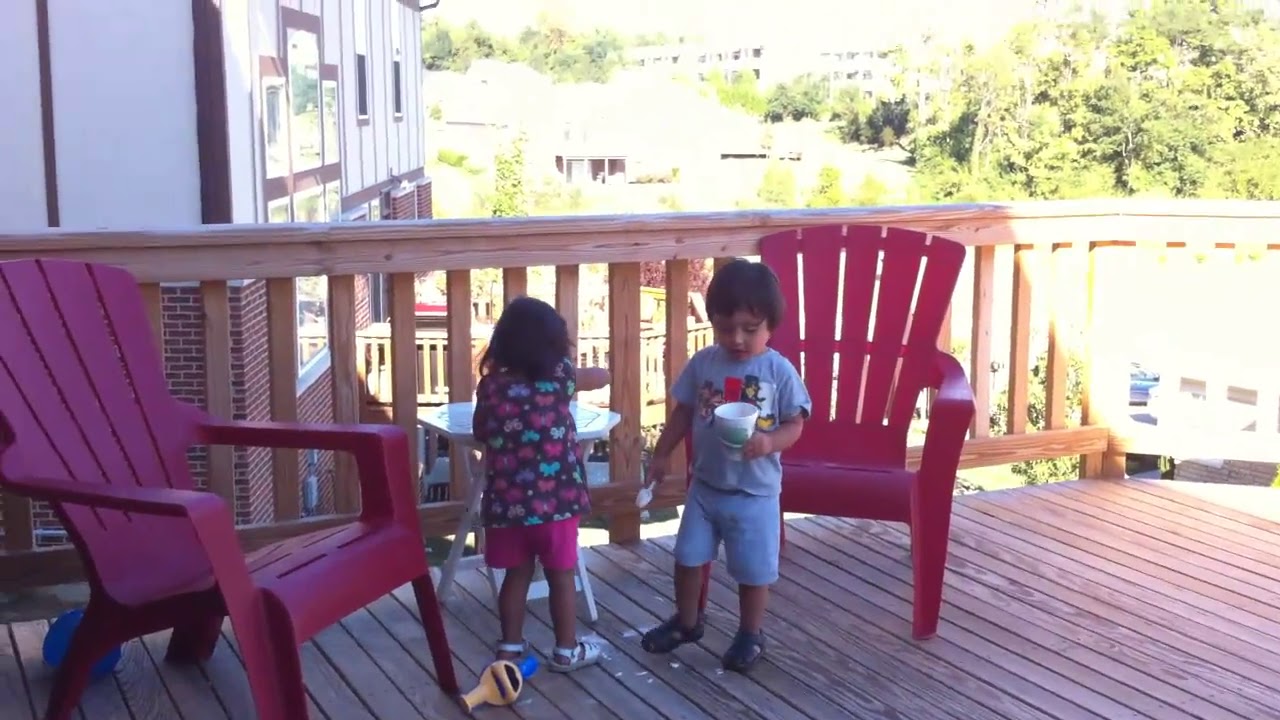This image captures a scene on a high, wooden deck adjacent to a white building with brown wood and brick accents. Two toddlers stand at the center—one boy and one girl. The boy, dressed in a grey t-shirt, grey shorts, and blue sandals, faces the camera, holding a white cup and a spoon. To his left stands the girl, her back to the camera, wearing a colorful shirt with a floral pattern and pink shorts, complemented by white sandals. She appears to be reaching towards her mouth, possibly eating something. The children are flanked by two large red plastic outdoor chairs that face toward the viewer. A small white round table stands in front of the girl, and at her left foot lies a yellow toy, while a blue toy is also visible on the deck. The deck is enclosed by a wooden fence, and additional buildings, along with tall trees, can be seen in the background, creating a picturesque, elevated scene.